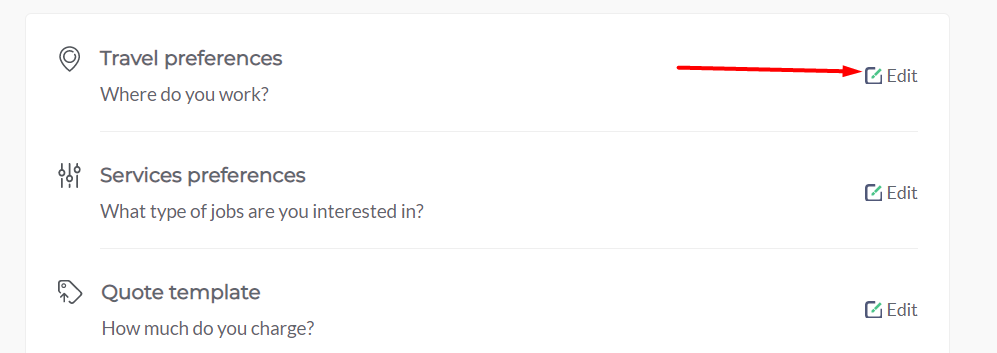This image is a cropped screenshot of an app's settings panel, showcasing a gray background with a large white rectangle overlaid on it. Visible gray areas are on the left, right, and top sides, while the bottom is cropped out. The "Travel Preferences" category is listed first, featuring the query "Where do you work?" with an "Edit" option on the right, highlighted by a prominent, narrow, and extended red arrow pointing to it. This arrow has been added to indicate the clickable area for editing.

Underneath, the "Service Preferences" section includes a prompt in light gray text: "What type of jobs are you interested in?" This section also has an "Edit" button on its right. Lastly, there is a "Quote Template" category asking "How much do you charge?" with an "Edit" option situated to its right. The overall layout and the added red arrow emphasize interactive elements related to customization within the settings panel.